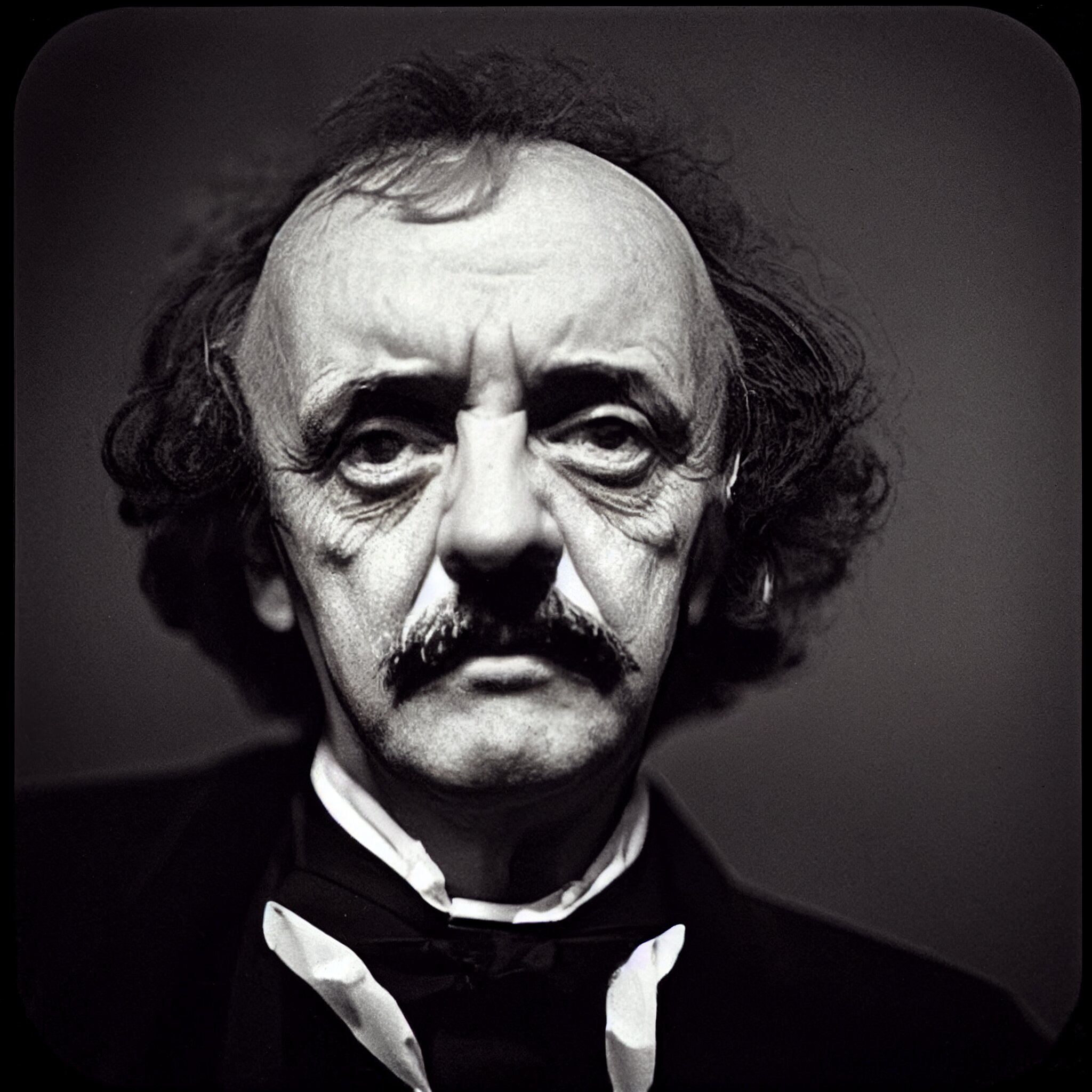This black and white photograph captures a man in his 80s with a prominent mustache that completely covers his upper lip. His dark hair is visibly receding, leaving him significantly bald on top, though he still has somewhat long, wavy hair that extends past his ears. There is no apparent gray in his hair, which appears curly towards the sides and back of his head. His forehead is wide, tapering down towards his chin, lending a distinctive shape to his facial features.

His eyes, which droop noticeably, are framed by large under-eye bags and deep wrinkles, especially between his eyebrows and at the corners of his eyes. These features give him a weary and melancholic appearance. He wears a white shirt adorned with a bowtie and is covered by a dark-colored jacket, typical of formal attire. The background is a light to medium gray, and the image is a perfect square, highlighting his upper body in a sharply contrasted, monochromatic palette. The overall expression on his face is neutral with a hint of sadness, contributing to the somber mood of the photograph.